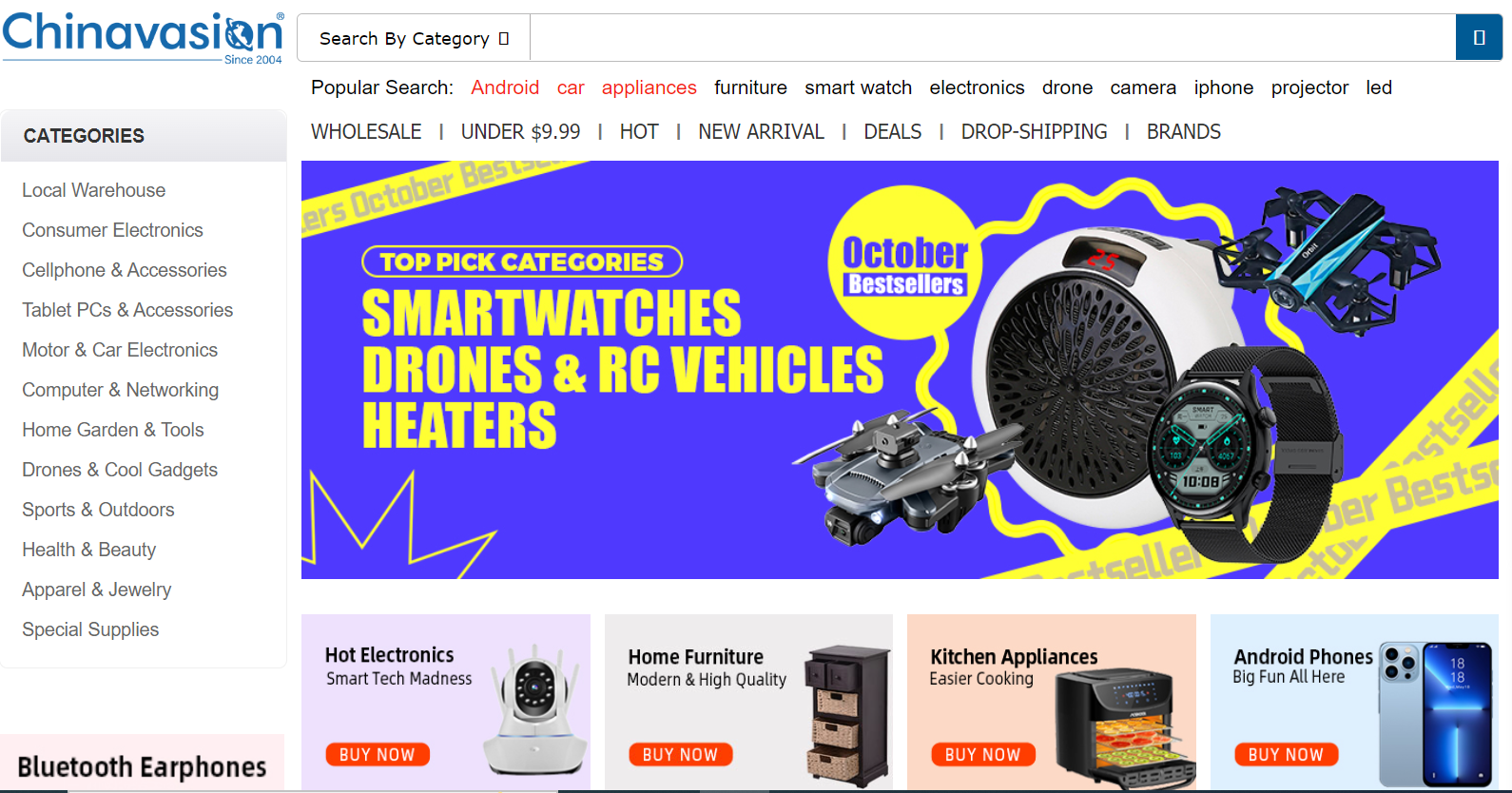Top search is China Evasion, showcasing a diverse range of popular categories. These include Android car appliances, furniture, smartwatches, electronics, drones, cameras, iPhones, projectors, LED lights, and wholesale products under $999. Highly sought-after items are highlighted as hot and new arrivals, including duos and drop shipping options. Featured brands and trending colors like blue and yellow, along with top categories such as smartwatches, drones, RC vehicles, and heaters, are prominently displayed. Specific searches also include yellow circuses and October bestsellers. Central to the display is a detailed list of categories organized by local warehouses and consumer electronics, encompassing cell phones, accessories, tablets, PCs, car electronics, computer networking, home gardening tools, eco gadgets, sports and outdoors gear, health and beauty products, and jewelry. Special supplies like Bluetooth earphones, hot electronics, and smart tech are also featured. Vibrant visuals marked by madness, red ovals, and a variety of cameras, home furniture, high-quality drawers, kitchen appliances for easier cooking, ovens, and smartphones, including large Android options and big phones, round off the search results, emphasizing a user-friendly "Buy Now" call to action.